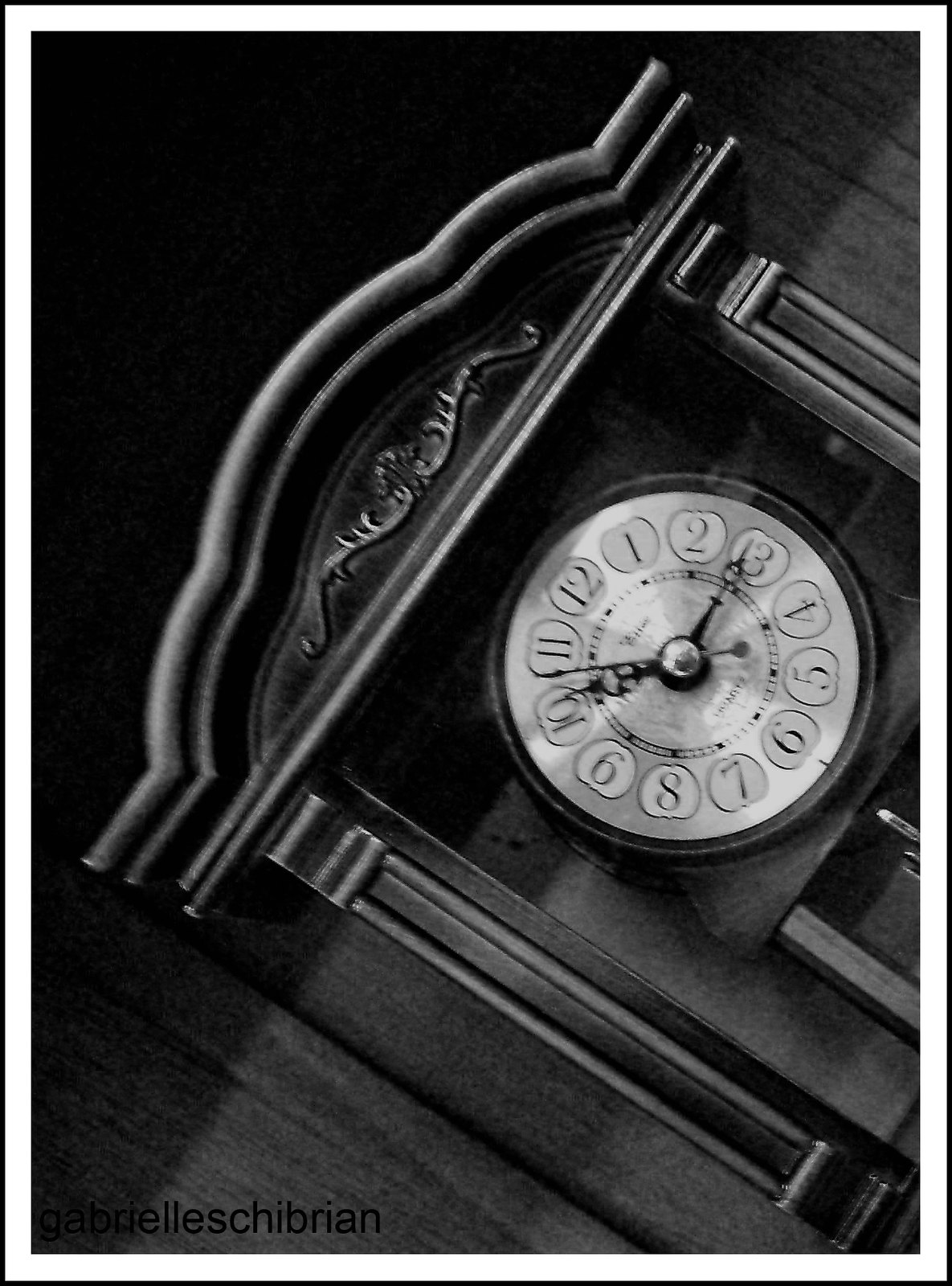In this black and white photograph, an old-fashioned clock stands as the focal point. The clock face, a weathered white, displays numbers from 1 to 12, each encircled by apple-shaped borders. The hands of the clock are intricately designed, ending at a central silver dot. Surrounding the numbers is a distinct black ring. The clock is encased in a dark wooden frame, complemented by an ornate design at the top. The backdrop features a wooden wall, casting a shadow along its upper edge, adding depth to the image. The photograph is taken at an angled perspective, giving a dynamic view of the clock. At the bottom left corner, there is text in an unreadable foreign language in black ink. A white border frames the entire image, enhancing its vintage charm.